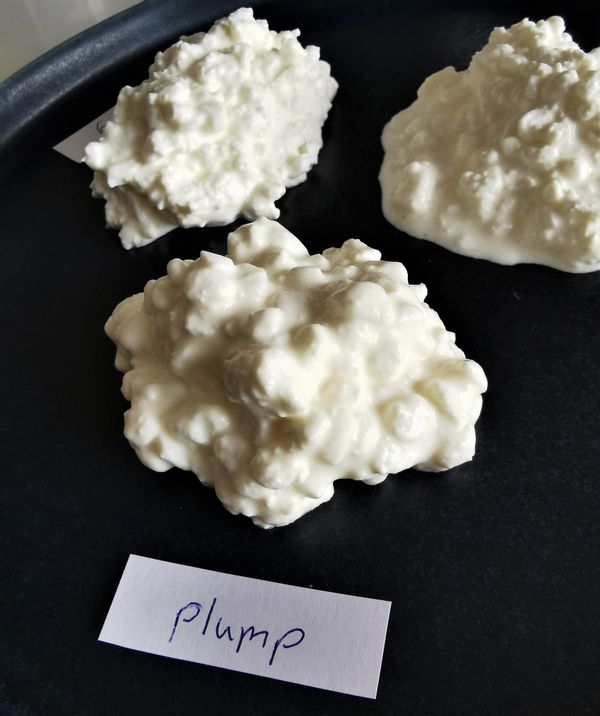The image depicts a black tray, possibly metallic or vinyl, with three conspicuous white clumps arranged in a triangular formation. These clumps have a consistency reminiscent of cottage cheese but appear more congealed, suggesting a hard white chocolate or mashed potato-like texture. The largest clump is positioned at the bottom center of the tray, prominently labeled with a handwritten piece of paper that reads "plump" in slightly uneven blue ink, where the initial 'P' is faint. Above this main clump are two smaller ones – the upper left clump has a label that appears to end with the letter "G," albeit partially obscured, and the label on the upper right clump is unreadable but presumably exists. The arrangement of these clumps and their distinct labeling indicate they might be part of a cooking test or experiment.